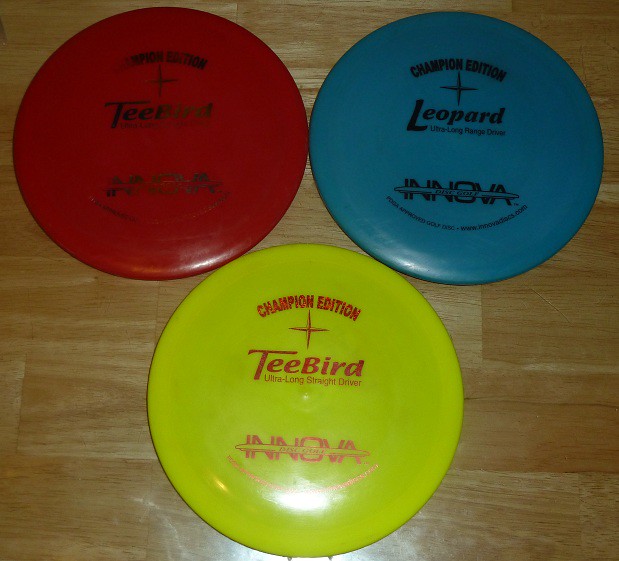The image showcases three frisbees arranged in an inverted triangular pattern on a red oak hardwood surface. The wooden grain runs horizontally from left to right. Each frisbee features identical designs but varies in color: a red frisbee on the top left, a blue frisbee on the top right, and a yellow frisbee in the bottom center. They are labeled "Champion Edition TeeBird" or "Champion Edition Leopard" and feature additional difficult-to-read text. All frisbees include the Innova logo, a white band, and a circular imprint at the bottom, although some text appears worn off or out of focus. A notable light source illuminates the lower part of each frisbee, highlighting the vibrant yellow one prominently. These frisbees are specially designed for frisbee golf, marked as ultra-long range drivers.